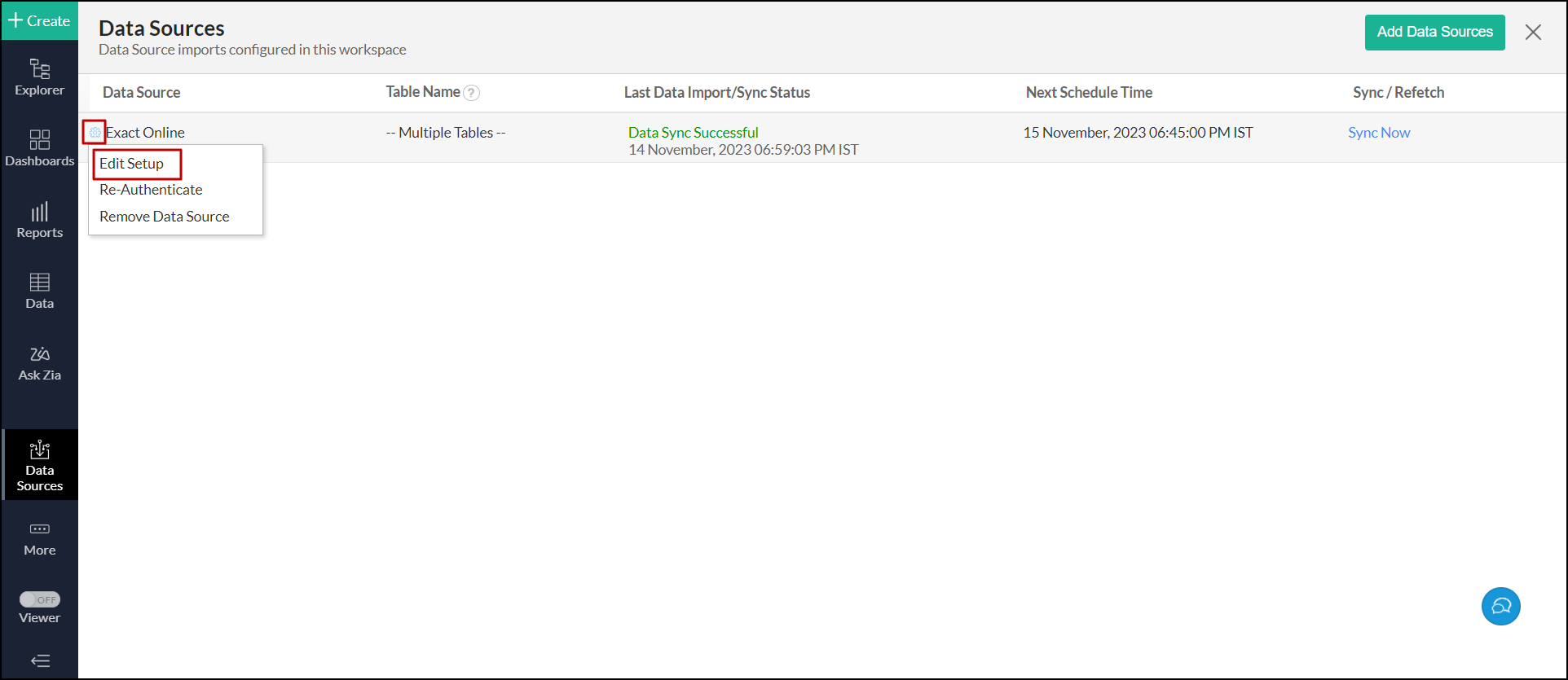This image depicts a detailed screenshot of a computer screen displaying a data management interface. On the left side of the screen, there is a vertical menu with a black background. At the top of this menu, in the upper left-hand corner, a prominent green rectangle features a white plus sign accompanied by the text "Create." Beneath this, there are eight icons, each with associated menu names listed in order from top to bottom: Explorer, Dashboards, Reports, Data, Ask Zia, Data Sources, More, Viewer, followed by three small hash marks.

Dominating the main section of the screen, the header "Data Sources" is prominently displayed. Additionally, the subtitle "Data Source Imports Configured in this Workspace" is visible. Directly below this, a table header comprises several columns labeled: Data Source, Table Name, Last Data Import, Sync Status, Next Schedule Time, Sync, and Refetch.

Within this table, there is a specific entry highlighted, labeled "Exact Online," distinguished by a red square next to it. Below this label, a contextual menu offers three options: Edit Setup (which is currently emphasized with a red rectangle around it), Reauthenticate, and Remove Data Source.

In the upper right-hand corner of the screen, a green rectangle labeled "Add Data Sources" is visible, providing an option for adding new data sources. Finally, a small blue circle is positioned in the lower right-hand corner of the screen, likely serving an additional functional purpose or as an interactive button in the user interface.